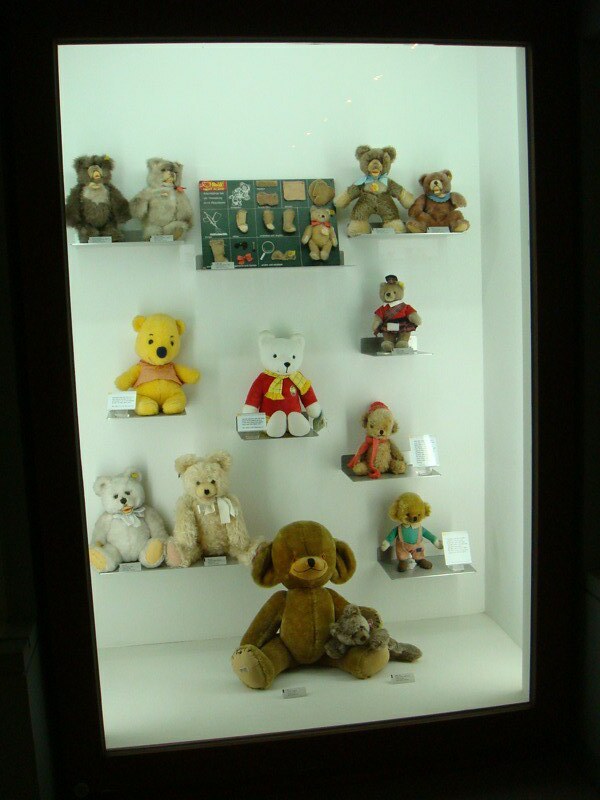The photograph showcases a display of vintage teddy bears arranged within a glass case that features a thick black rectangular border. The interior is illuminated with a white backdrop and floor. Shelves arranged on the back wall hold the bears, with the top two shelves each hosting two bears, while the remaining shelves feature one bear each. At the center of the display is a green board displaying teddy bear parts. Notable in this collection is a packaged bear kit with unreadable text. 

On the floor sits the largest bear, cradling a smaller bear on its right leg, reminiscent of a child cuddling with a parent. Several bears are adorned with clothing: one wears a yellow scarf and red shirt, another resembles Winnie the Pooh with a peach shirt, while others have blue neck accessories or tiny hats. A particularly notable bear at the bottom is dressed most elaborately in a bluish-green shirt, overalls, and possibly socks. The display is diverse, featuring various colors, shapes, and sizes of bears, each accompanied by small, unreadable informational plaques.